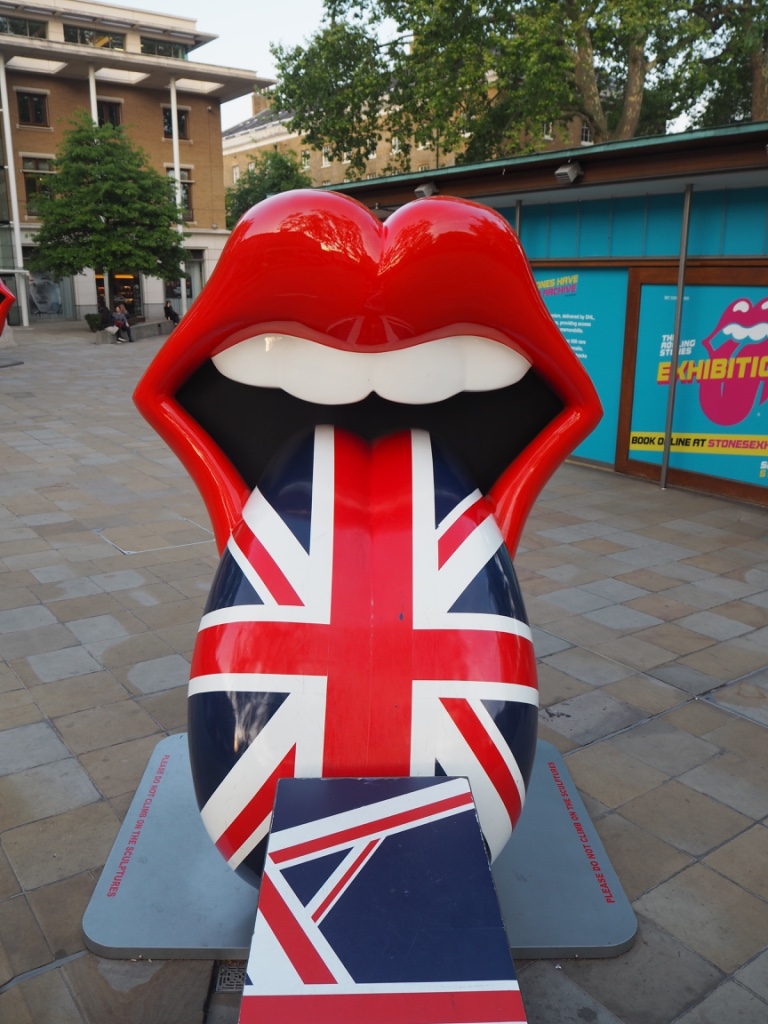The image captures a close-up of a three-dimensional statue based on the iconic Rolling Stones mouth and tongue logo. The art piece features red lips, four white teeth, and a tongue that prominently displays the Union Jack pattern—red and white lines on a dark backdrop. The tongue stretches out towards the viewer, partially obscuring a cardboard box adorned with a similar Union Jack design leaning against its tip. The entire statue is mounted on a light gray base, set on a tiled outdoor patio. In the background, there are lightly colored tan brick buildings and trees, with people seated on concrete benches. A bright blue billboard to the right reads "The Rolling Stones Exhibition - Book Online" but is partially obscured by the statue. Additional text on the pink Rolling Stones logo against the blue background is visible but unreadable due to obstruction. The scene suggests that the artwork is part of an exhibition in London.